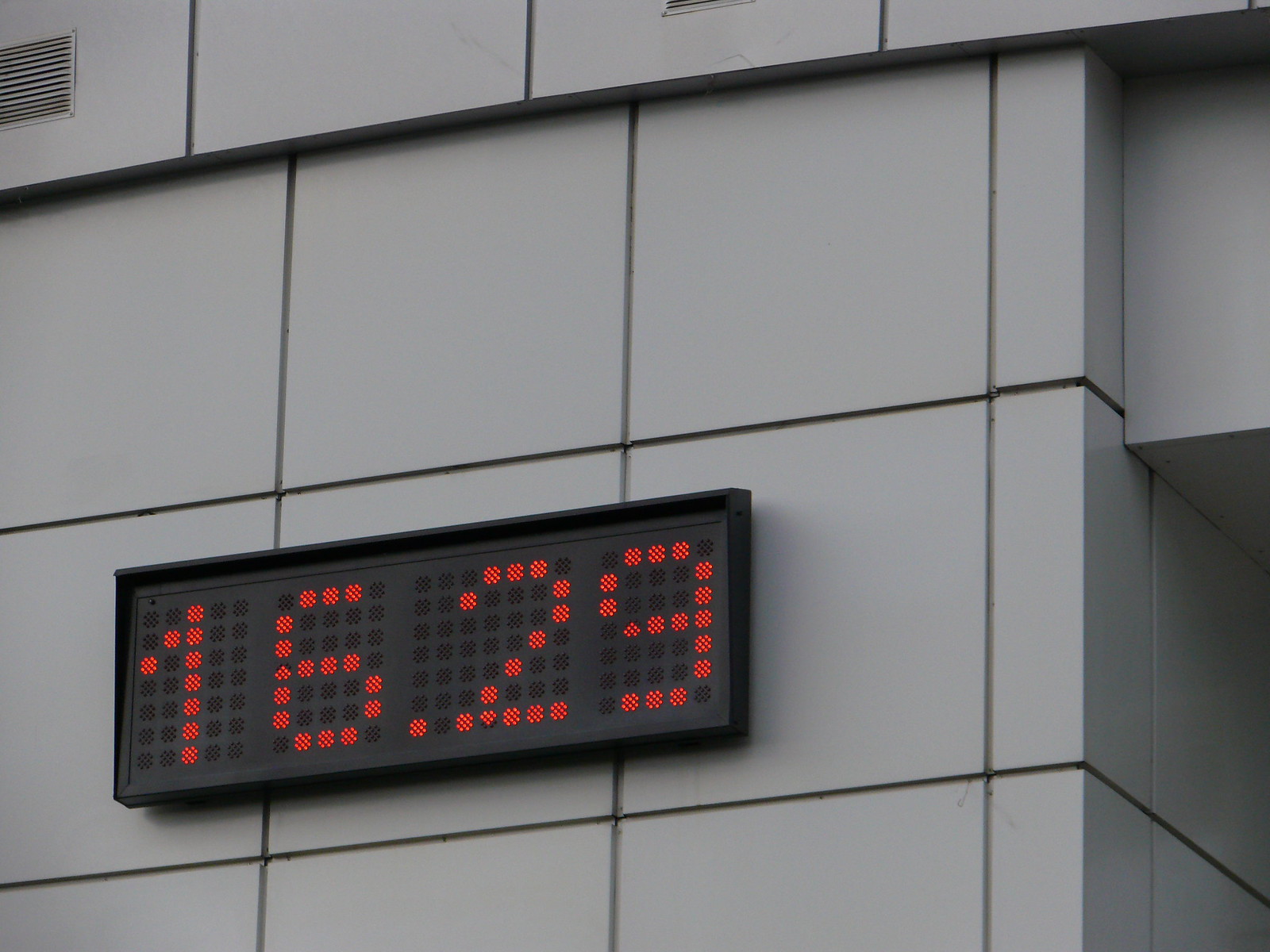This color photograph shows the side of a building made of grey concrete square tiles neatly fitted together, each approximately four inches by four inches, with black grout running between them. Dominating the image is a large black rectangular digital clock positioned in the lower-left to center part of the photo. The clock displays the time 16.29 in bright red numerals. The clock’s design features thin edges extending slightly past the main display, creating a subtle 3D effect with a slight shadow underneath. In the top left corner of the image, there is a small silver vent, while the right side of the frame shows part of an overhang, suggesting an entryway.